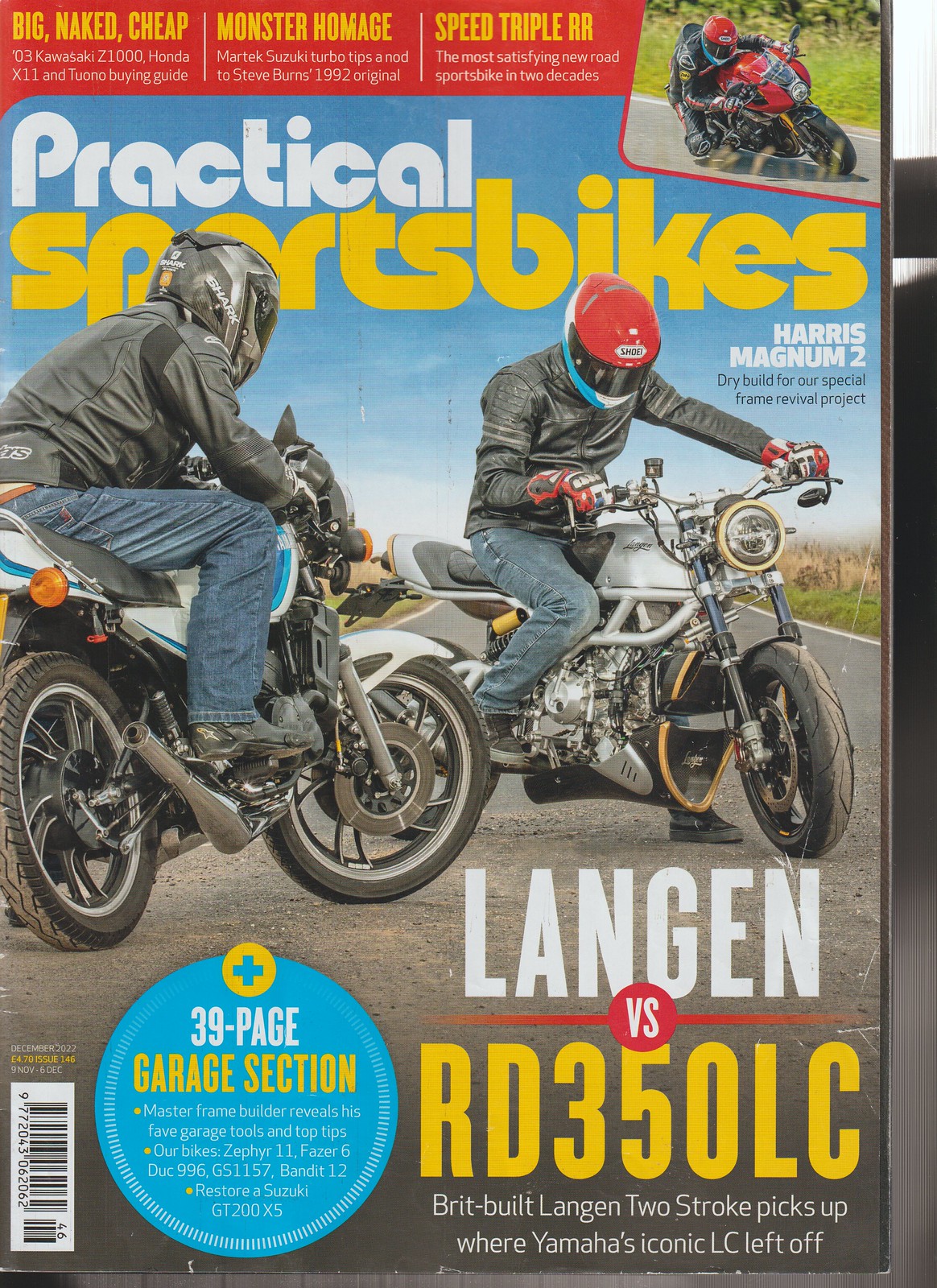The cover of the magazine titled "Practical Sport Bikes" prominently features two motorcycles ridden by men on a highway with a blue sky backdrop. The rider on the left is on a white motorcycle with blue stripes, black tires, and a chrome exhaust, wearing blue jeans, a black leather jacket, and a black and gray helmet. The other rider, positioned front-center, is on a mostly gray motorcycle with a yellow circle around the headlight, also in blue jeans and a black leather jacket, but with a red helmet. The asphalt is black and the overall setting emphasizes sports biking. Visible taglines include "Big Naked Cheap," "Monster Homage," and "Speed Triple Bar," with highlights on Kawasaki Z1000, Honda X11, and Turbo Tips. At the bottom left, there is a vertical barcode, and on the bottom right, it reads "Langen vs RD350 LC," noting that the Brit-built Langen two-stroke picks up where Yamaha's iconic LC left off. Additional small text references articles and other features, including a mention of Steve Burns' 1992 original and Harris Magnum II Drive Builds for a Special Frame Revival Project.